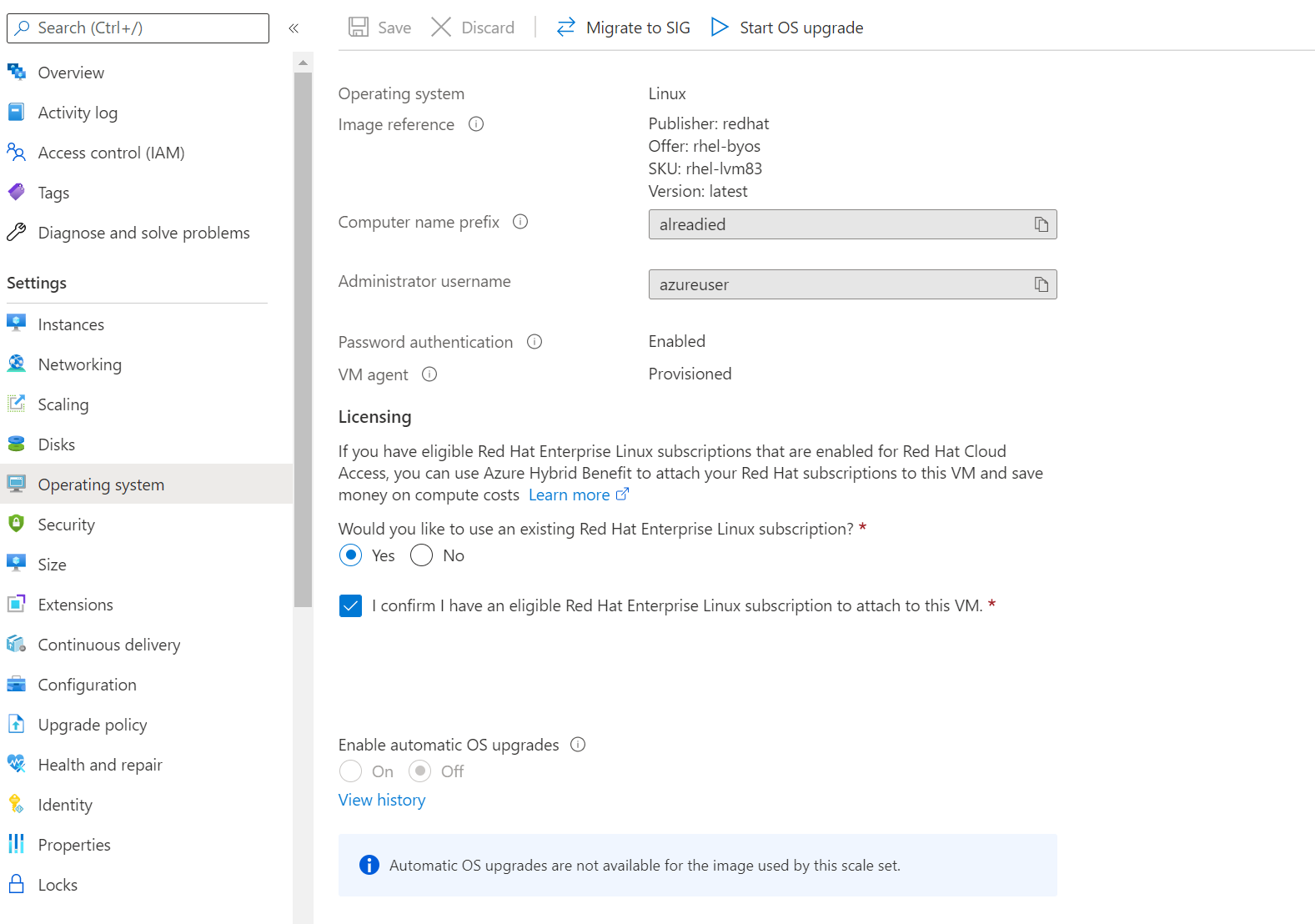The image displays a screenshot of a computer screen showcasing a detailed interface, likely an administrative panel or dashboard for managing cloud resources. At the top of the screen, there is a search bar with an icon indicating the shortcut "Control + /."

On the left side of the screen, a vertical sidebar is populated with labeled icons for different management sections. The sections listed, in order from top to bottom, include:
- Overview
- Activity Log
- Access Control (IAM)
- Tags
- Diagnose and Solve Problems (represented by a wrench icon)
- Settings
- Instances
- Networking
- Scaling
- Disks
- Operating System
- Security
- Size
- Extensions
- Continuous Delivery
- Configuration
- Upgrade Policy
- Health and Repair
- Identity
- Properties
- Locks

A vertical scroll bar suggests there are more sections that can be viewed by scrolling up or down.

In the main central area of the screen, more specific configuration settings are visible. This section includes areas for:
- Operating System
- Image Reference
- Computer Name Prefix
- Administrator Username
- Password Authentication
- VB Agent
- Licensing area (with an option marked as "Yes")

The layout and labels indicate a comprehensive and detailed interface, likely used for configuring and managing various aspects of a cloud computing environment.